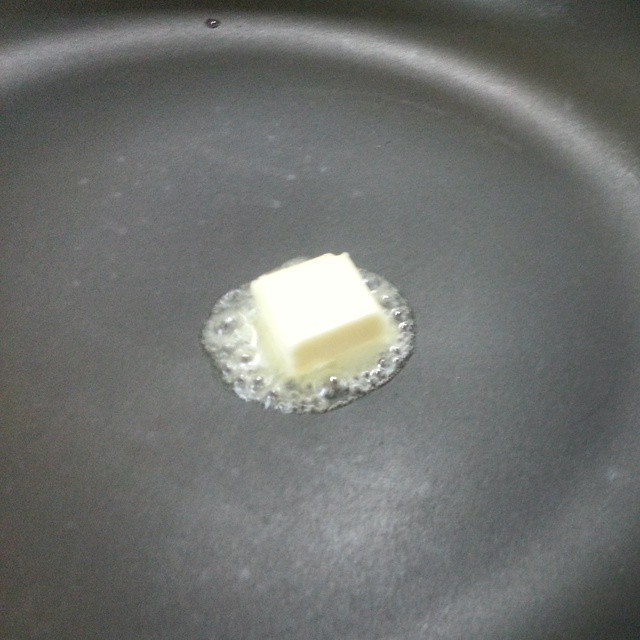This image features a close-up view of a small, light yellow square pad of butter, approximately one inch by one inch and a quarter-inch thick, set in the center of a black non-stick frying pan. The butter is partially melting, creating a circular, translucent melted area tinged with yellow around its edges. Tiny bubbles are forming in this surrounding melt, indicating that the pan, which catches light from above, is already hot or heating up. Scattered near the outer edges of the pan, a solitary drop of water hints at the pan's temperature. The entire scene captures the precise moment where the butter begins to succumb to the heat, with the bubbling action emphasizing the pan's readiness for cooking.